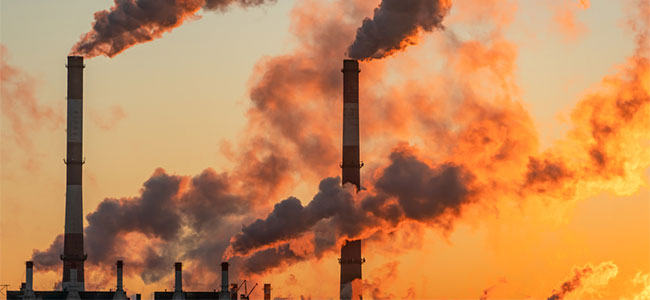The photo captures an industrial scene dominated by multiple smokestacks from manufacturing plants or oil refineries, set against a vibrant sky at either sunrise or sunset, characterized by hues of orange, yellow, and purple. In the foreground, two tall smokestacks stretch skyward, standing prominently at approximately three stories high and making up about three-fourths of the image. These smokestacks, along with at least four or five smaller ones situated closer to a factory roof, are emitting thick, orange-gray to black smoke that nearly obscures the sky. The dense fumes, billowing vigorously, create a stark contrast with the scant patches of blue visible in the top corners of the image. The factory itself remains indistinct, with the focus solely on the pollution dominating the scene.